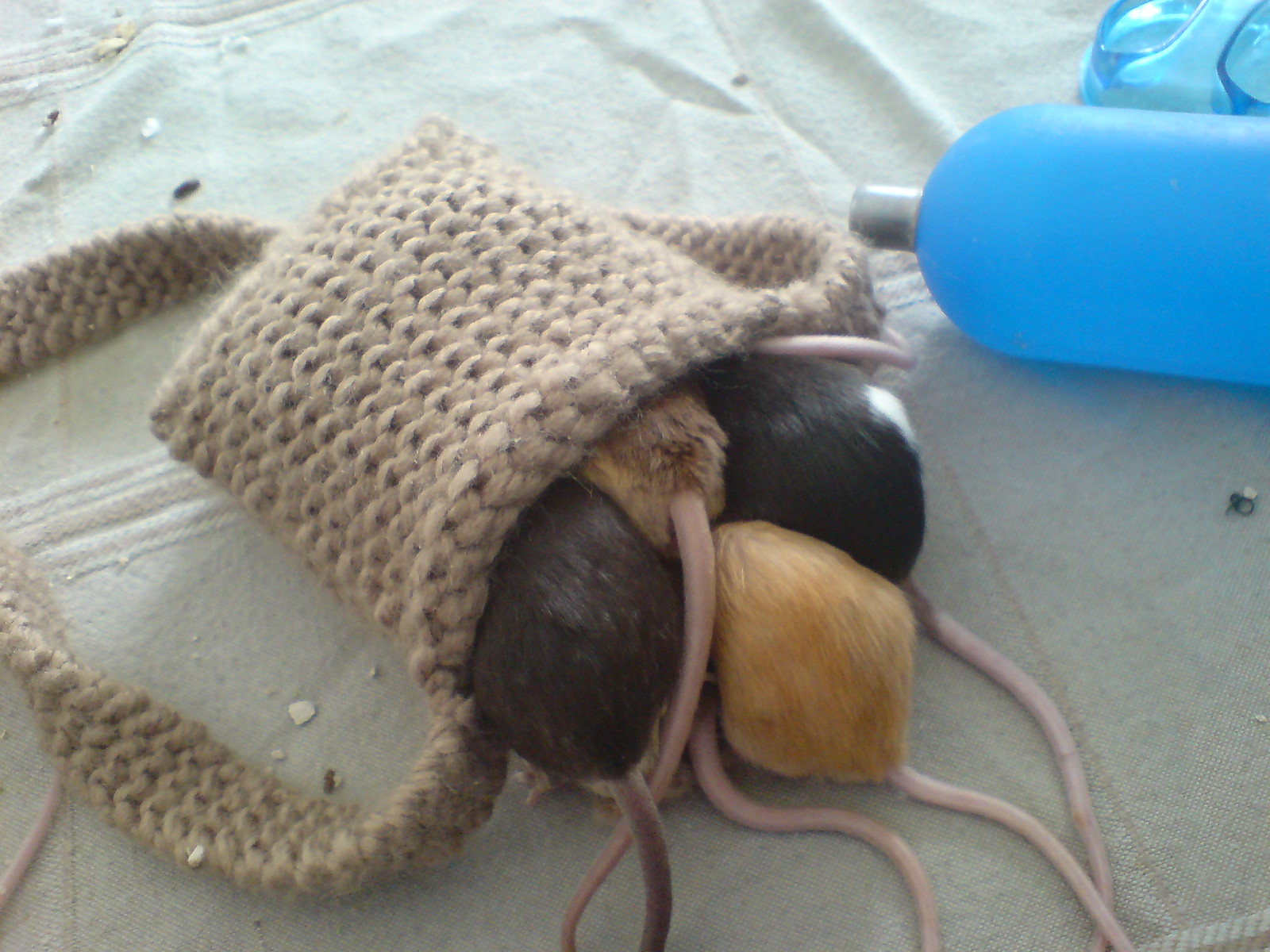This brightly lit horizontal photograph features a light beige, possibly burlap or canvas, fabric laid out as the background. In the upper right corner, a blue plastic bottle with a silver metallic cap lies on its side, accompanied by another blue, transparent container beside it—possibly a glasses case or a mask holder. 

The center of the image is dominated by a small, tan, crocheted or knit pouch with a long strap. Inside this pouch, several rodents are nestled, displaying only their rear ends and tails. The rodents have pink, hairless tails, and their fur ranges in color: two are black, one has a white patch, another is medium brown, one is tan, and another is a lighter blonde or tan shade. There are at least five to six tails visible, suggesting a varying number of rodents, though not all their bodies are fully distinguishable. Crumbs or rat droppings are scattered on the fabric, adding texture and indicating the presence of the rodents.